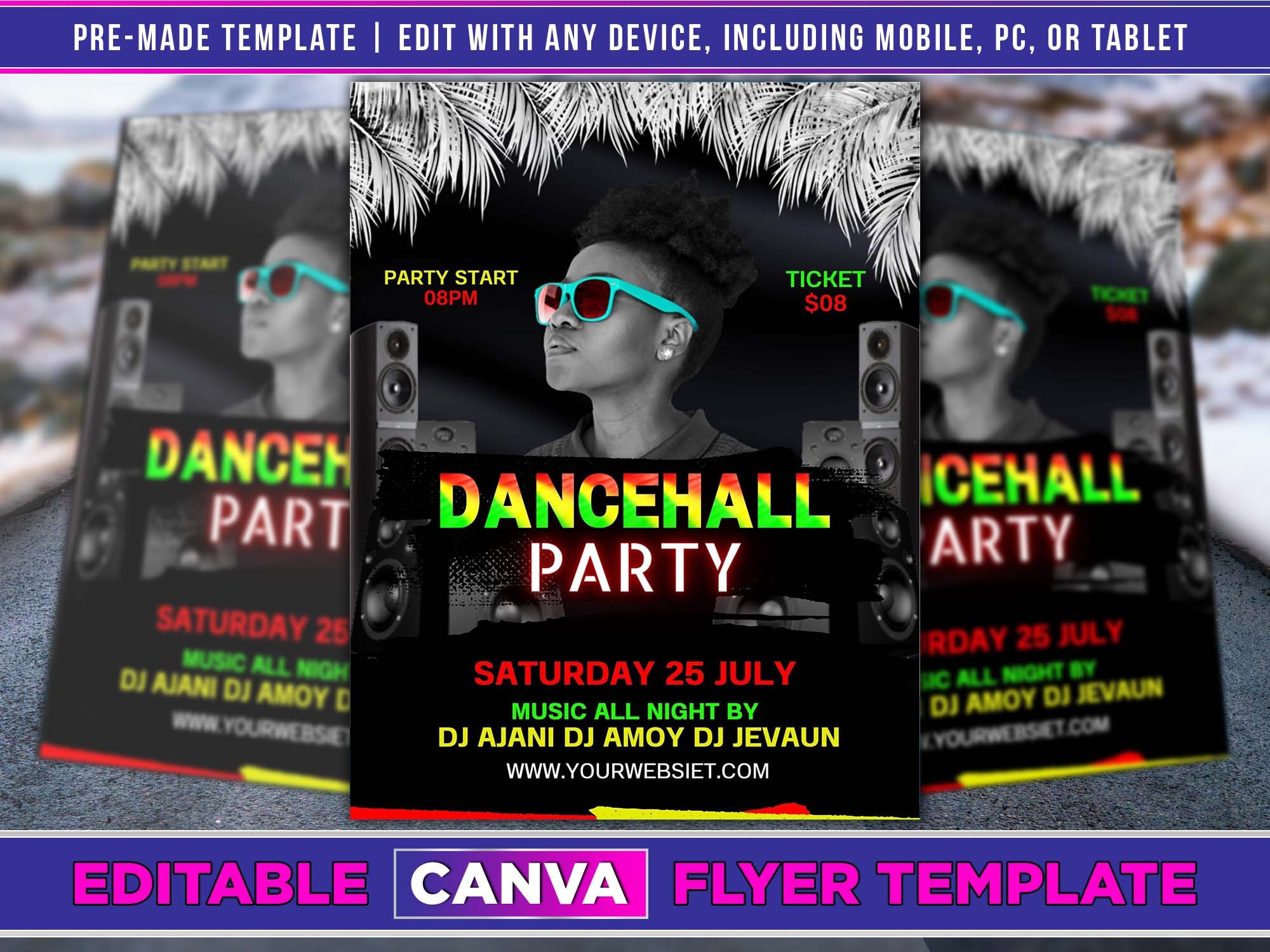This image showcases an advertisement featuring a poster centered between two blurred duplicates. The poster, set against a black background, promotes a "Dance Hall Party" on Saturday, July 25th. It highlights that music will be provided all night by DJs Ajani, Amoy, and Javon, and includes the website www.yourwebsite.com for more details. Central to the poster is an image of a black woman with short curly hair styled into a shaved afro. She is adorned with turquoise sunglasses with red lenses and earrings, looking to the right. There are black speakers around her. Additionally, the flyer details that the party starts at 8 PM and tickets are $8. Surrounding the main content is a top and bottom border in purple; the top border states in white letters, "Pre-Made Template. Edit with any device, including mobile, PC, or tablet," while the bottom border declares in pink letters, "Editable Canva Flyer Template."